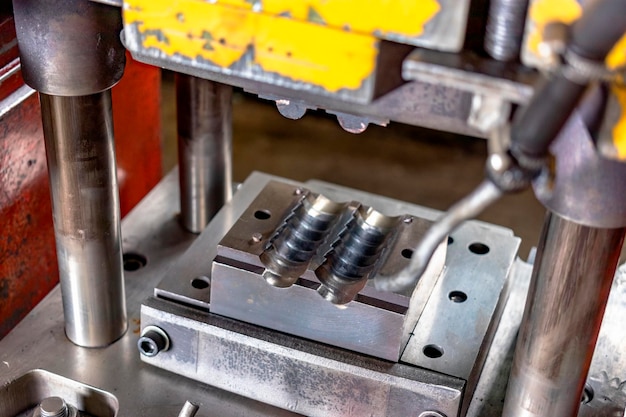The image depicts an old, well-used mechanical press situated in what appears to be an industrial or workshop setting. Central to the image are two metal poles emerging from a flat surface, extending upward and supporting additional metal components at the top. Once predominantly yellow, the paint is now worn, giving the machine a rugged, aged appearance. The core mechanism features a cylinder-like structure that likely functions by applying pressure downward, akin to a press designed to match up with grooves on a thick, silver rectangular base and a grooved square piece. The machinery's various parts include holes, divots, and ridges that suggest precision alignment. Shiny metallic surfaces gleam under good lighting, and a toolbox is visible on the left side, further emphasizing the workshop environment. Red and yellow paint marks add to the detailed, utilitarian aesthetic of the setting.